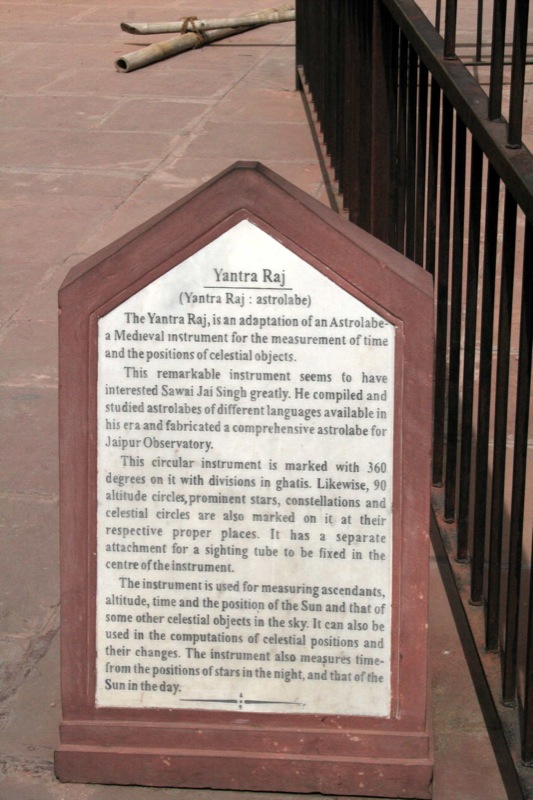In this image, set on a brick-tiled surface, we see an intriguing outdoor setting captured in the middle of the day. At the top of the frame, a couple of sticks are lying down, while a guardrail is visible on the right side, adding context to the location. Dominating the center of the image is a prominent statue or monument inscribed with the words "Yantra Raj." This remarkable instrument is an adaptation of an astrolabe—a medieval tool used for the measurement of time and the position of celestial objects. Historically significant, the Yantra Raj fascinated Sawai Jha Singh, who compiled and studied astrolabes from various languages of his era to create a comprehensive astrolabe for the Jodhpur Observatory.

The circular instrument is meticulously marked with 360 degrees, divisions on gaddis, and indications of 90 altitudes, prominent stars, constellations, and celestial rings. The setup also features a separate attachment for a sighting tube, positioned at the center of the instrument. The astrolabe serves multiple functions, including measuring ascendance, altitude, time, and the positions of the sun and other celestial bodies. Additionally, it can compute the positions of celestial objects and their changes over time, and determine time based on the position of stars at night and the sun during the day.

The color palette of the scene includes shades of brown, white, black, off-red, and gray, adding to the historical and scientific ambiance of the setting. This detailed depiction showcases the Yantra Raj astrolabe's significance and its intricate design, reflecting the rich heritage and astronomical advancements of its era.